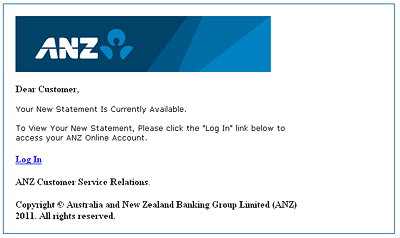The image is a rectangular box predominantly featuring a white background. The top portion, which takes up about two-thirds of the image's width, contains a blue box that spans from left to right. The blue box consists of varying shades of blue and displays the white letters "A" and "Z." Adjacent to these letters, there is a lighter blue 'ampersand' symbol. 

Following the blue box, the content is displayed in a format similar to an email. It starts with a bolded greeting: "Dear Customer," followed by the message: "Your new statement is currently available to view. To access your new statement, please click the login link below to access your A and Z online account." 

Beneath this message, a blue hyperlink with the text "Log In" – where "Log" and "In" are capitalized and separated – invites users to log in. Below this link, the text "A and Z Customer Service Relations" is bolded, followed by a copyright notice: "© Australia and New Zealand Banking Group Limited (A and Z) 2011. All rights reserved." 

The entirety of the text and elements rests on a clean white background, except for the blue box at the top. This image appears to be a screenshot of an email or webpage related to A and Z banking services.